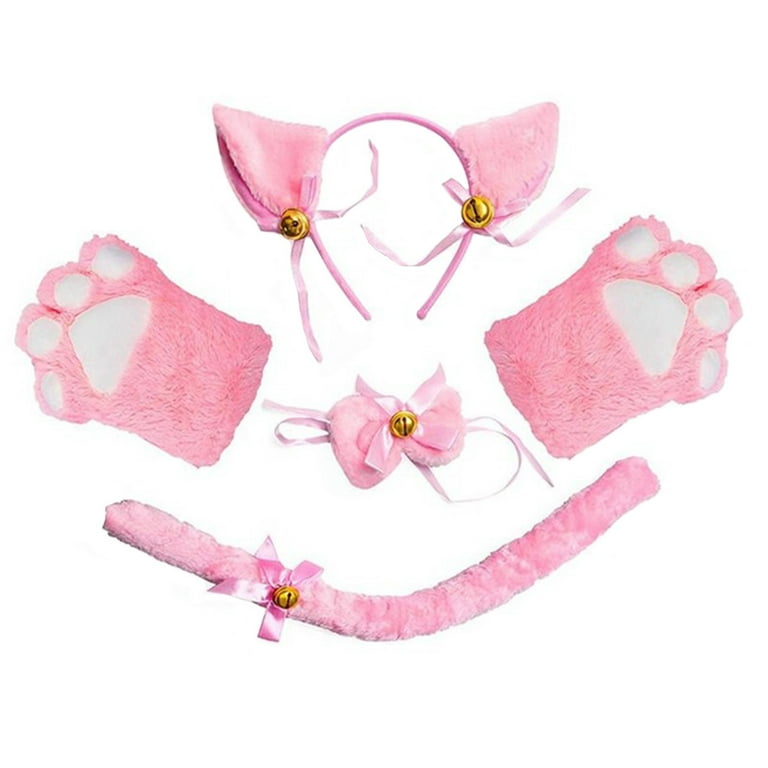This detailed product image, likely from a catalog or online store, features a five-piece pink kitten costume set designed for dress-up roleplay, cosplay, or Halloween. The set includes a pink headband adorned with furry ears, a pink strap-on bow tie collar, two pink gloves shaped like animal paws with white pads, and a pink plush tail. Each accessory is accented with golden bells and pink bows, adding a charming detail. The items are carefully arranged on a plain white background, with the headband at the top, the gloves on either side, the collar in the center, and the tail at the bottom, giving a clear view of each piece in the pink cat ensemble.